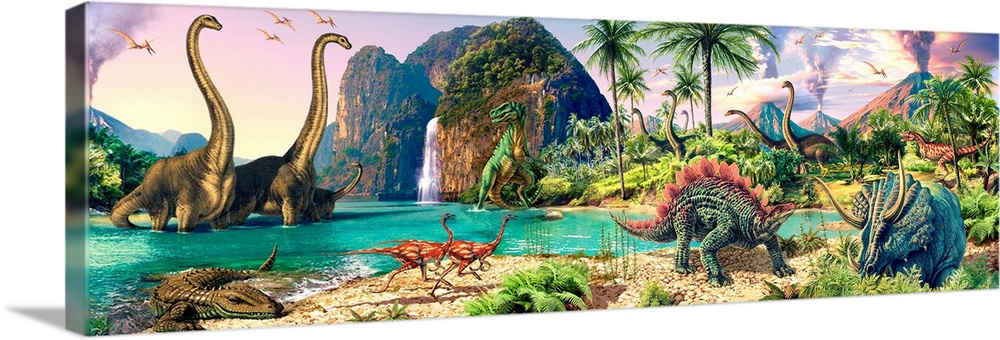The image showcases a detailed and vibrant canvas print, presenting a prehistoric scene teeming with dinosaurs. The composition spans horizontally, capturing a lush, Eden-like jungle. A serene waterfall cascades in the background, framed by towering, tree-capped mountains. To the right, multiple volcanoes billow with smoke, adding a sense of dramatic tension. In the foreground, a dark green Triceratops and a lighter green Stegosaurus stand near the lush, tan shore. An alligator-like creature, sporting a brownish-green hue, crawls from the water while a family of grayish-brown Brontosaurus wades through the picturesque, teal water. Tiny, bird-like Gallimimus dart around, reminiscent of roadrunners. High above, pterodactyls soar, adding movement to the sky, while a bright green T-Rex with a yellow underside stands prominently at the center, eyeing the scene. The landscape, dotted with verdant greenery, shrubs, and rocky outcrops, brings the prehistoric world to life with an astonishing level of detail.